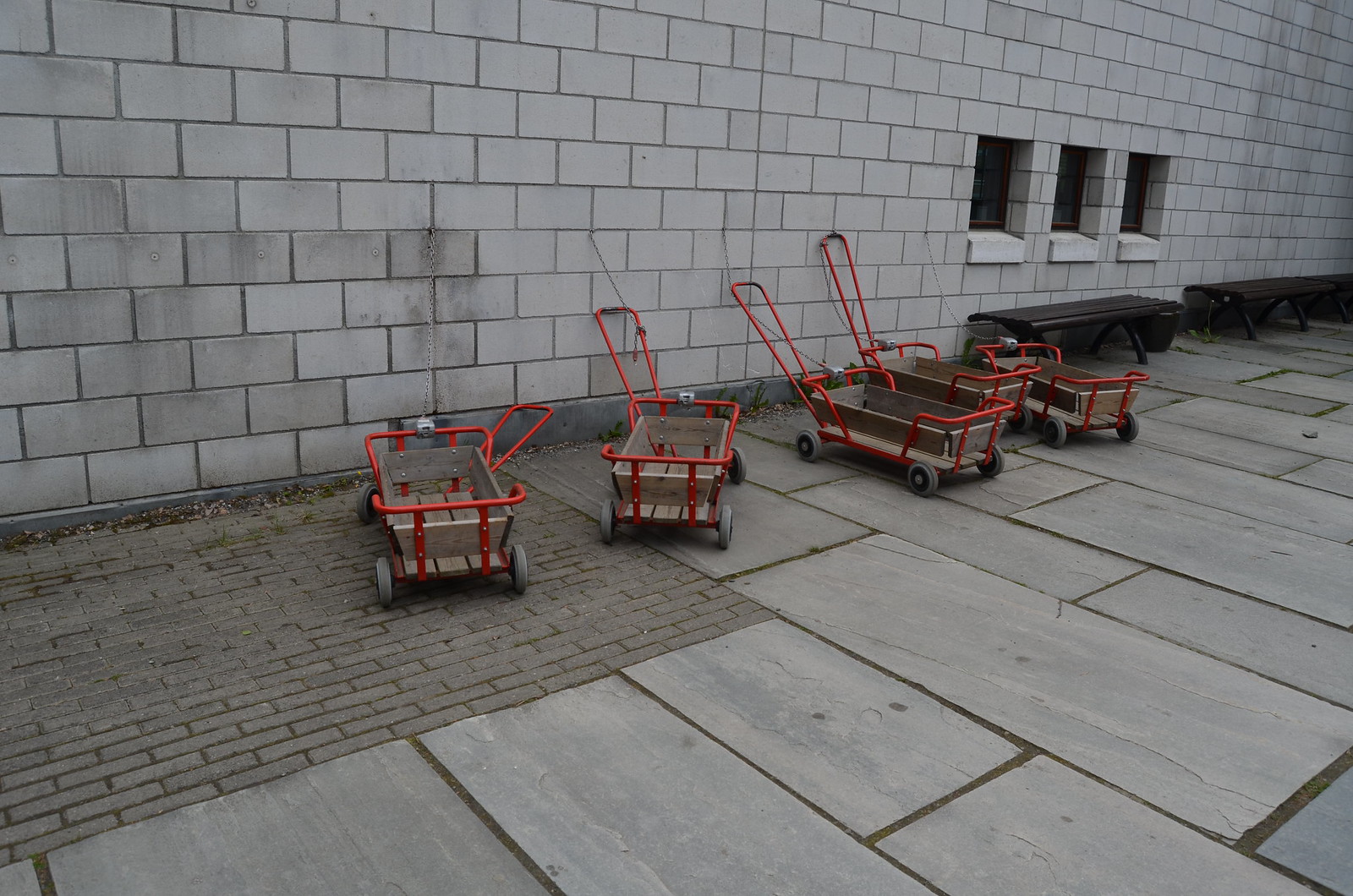This image depicts an outdoor courtyard featuring distinctive flooring comprising large rectangular tiles, with a small section on the left-hand side composed of small gray bricks arranged in a square-like shape. Five miniature wagons stand prominently in the scene, each with a bright red metal frame, solid gray rubber wheels, and a square wooden base made from gray wood. These wagons have sturdy rails and looped handles that extend up and down, showing they are designed for pulling and transporting items or children. To the right, there are two long, black flat benches without backs situated against a light gray brick-styled wall. Above the benches, three rectangular windows are evenly spaced across the wall, completing the background setting of this courtyard area.